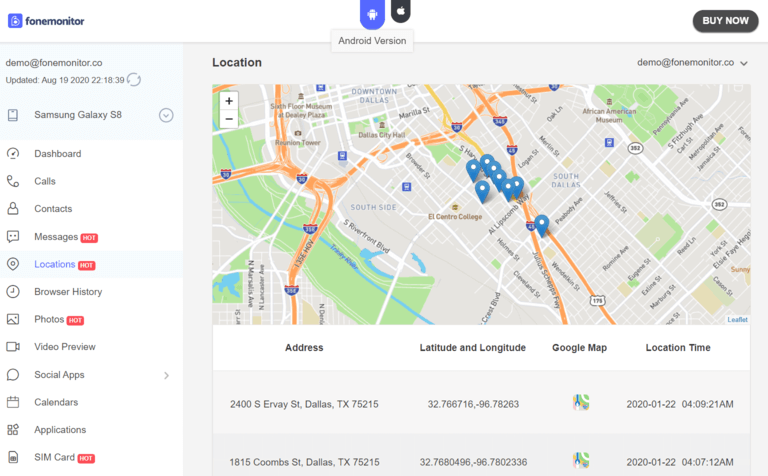This image displays a detailed screenshot of a mobile monitoring application interface on what seems to be a cellphone screen. In the top-left corner, "Phone Monitor" is written in black text, accompanied by a blue square. To the right, there is a black button labeled "Buy Now."

Centrally within the image are two small banners: one blue banner displaying a white robot icon and another black banner displaying a white Apple logo. On the left-hand side, there is a vertical blue-topped bar that reads "Demo" followed by "Phone Monitor," and a timestamp indicating "Updated August 19, 2022, 18:39." The device in use is noted to be a Samsung Galaxy S8.

Beneath this, there is a list of monitoring options on a white background, including: Dashboard, Calls, Contacts, Messages, Locations, Browser History, Photos, Video Preview, Social Apps, Calendars, Applications, and SIM Card. Notably, the options for Messages, Locations, Photos, and SIM Card are marked with a red "HOT" label in white text and all caps.

On the right side of the image, set against a grey background, is the title "Location" above a map from Google Maps. This map displays several blue location markers with white dots clustered around an area in Texas. Below the map are two addresses: "3024 S R L Thornton Fwy, Dallas, Texas, 75224" and "1815 S Ewing Ave, Dallas, Texas, 75216."